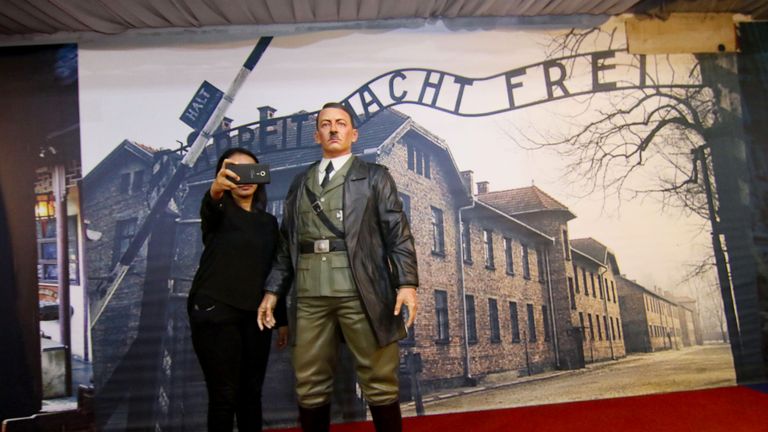This photograph captures a poignant scene set in what appears to be a museum or exhibit dedicated to the Holocaust. The central figures are a woman dressed entirely in black, taking a selfie with a wax figure of Adolf Hitler. The woman is holding her camera phone in front of her face, obscuring it from view. Hitler's wax figure is strikingly lifelike, dressed in his characteristic military uniform complete with a black leather jacket, an olive green military garb, a belt, and a black strap from shoulder to belt. They are positioned in front of a black-and-white backdrop featuring old brick buildings and a gate, reminiscent of a concentration camp. Partially obscured signage above, which seems to spell out something like "ARBEIT MACHT FREI," adds to the somber atmosphere. An emergency barrier arm for traffic control is also visible in this detailed background, along with a hallway leading outdoors. The photograph, devoid of text, is an indoor shot that aims to evoke the grim history of the Holocaust.